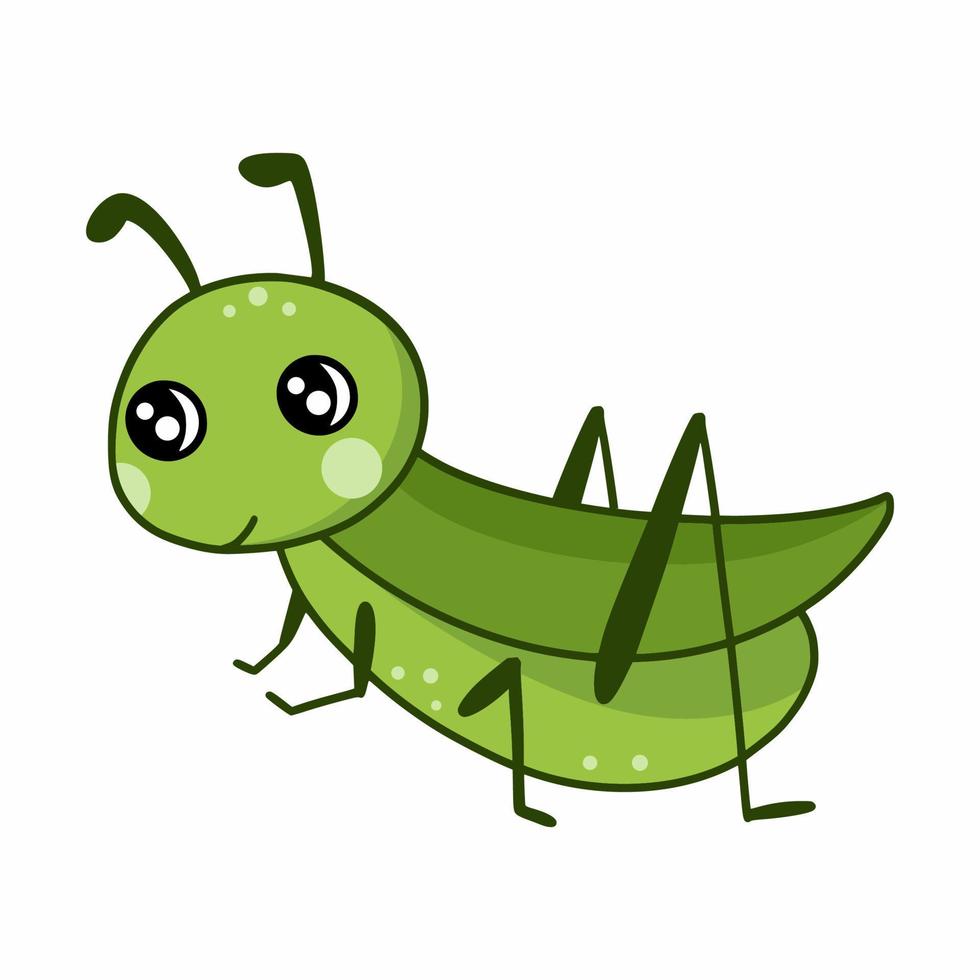The image is a color clip art of a simplistic, childlike green grasshopper against a white background. The grasshopper, which is light green with darker green antennae, has an oval face featuring large black eyes with white crescent moons on the right side and two white dots inside the black. It has small, circular white cheeks and a tiny black line for its smiling mouth. The head is topped with three faint white dots. The grasshopper's body, reminiscent of a cucumber, is two-toned with a darker green top section and a lighter green bottom section that is dotted with white. It has five visible legs: two short front legs, an additional shorter middle leg, and two large, prominent back legs. The overall aesthetic is cute, cartoony, and simplistic, with the grasshopper's body turned to the left while its face looks forward, and a wing shaped like a leaf contributing to its charming appearance.